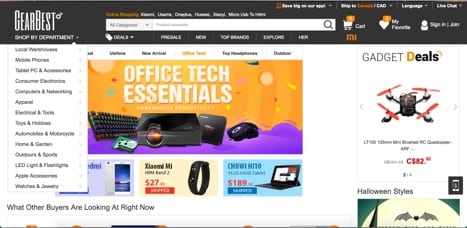The image depicts a section of the GearBest website. The dark-colored top navigation bar, which appears black, spans the width of the page. On the upper right-hand side, there are options for selecting the website's language and signing in. The center-justified search bar is prominent in this top bar, just to the right of the GearBest logo and the "Shop by Department" menu.

Directly below the search bar is a horizontal menu featuring various categories. Additionally, on the left side of the image, there is a vertical menu that lists options such as "Tablet PCs," "Accessories," and "Computer Networking."

The main focus of the webpage is a central visual showcasing "Office Tech Essentials," featuring images of a keyboard and a projector. This section draws the viewer's attention towards office-related tech products available on the site.